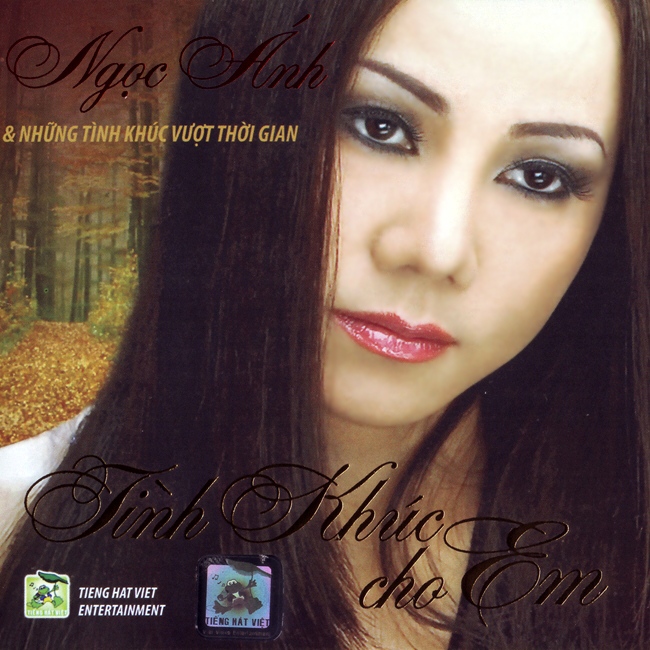The image is a full-color depiction that appears to be an album or CD cover. It features a close-up portrait of a young Asian woman, possibly in her mid-30s, with long dark brown hair and striking bright red lipstick. She's adorned with elaborate makeup, including pronounced eyeliner that enhances her pretty brown eyes. The background showcases a wooded forest scene, capturing the essence of a fall daytime with vibrant foliage. Text in Vietnamese covers parts of the image, indicating it might pertain to the Vietnamese entertainment industry, as suggested by the "Viet Entertainment" label at the bottom. This visual context implies that the woman could be a singer, posed elegantly amidst the natural setting, although this can't be confirmed definitively.